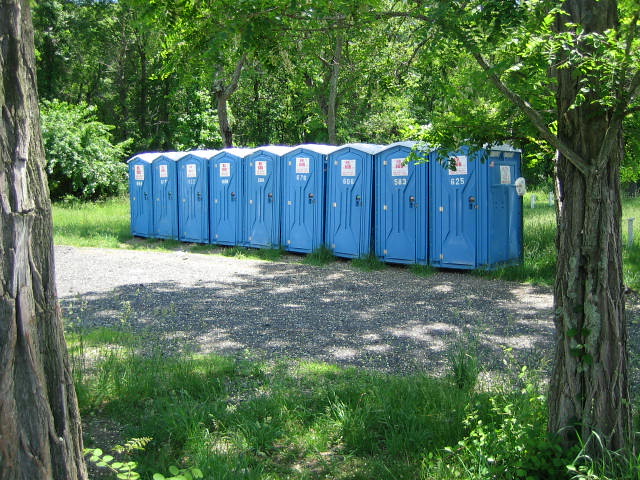In this photograph taken on a sunny spring or summer day in a forested area, a row of nine blue port-a-potties is prominently featured. These portable restrooms are lined up along a gray gravel path, each one labeled with unreadable white numbers on the doors and bearing a small, indistinct white sign. A strip of green grass lies between the gravel path and the camera's viewpoint. Flanking the viewpoint, two large trees with brown trunks stand in the foreground. The scene is set against a backdrop of dense, vibrant foliage and numerous trees, suggesting the location is a park or nature reserve, teeming with lush vegetation. The clarity of the sunlight adds a fresh, inviting ambiance to the image.